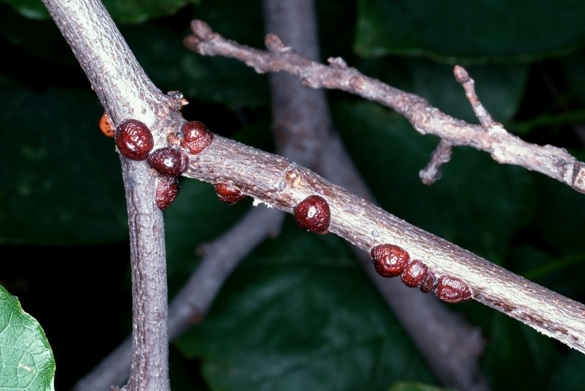In this nighttime nature photograph, the focus is on a slender tree branch adorned with peculiar red growths, possibly small snails or some form of insects. These red bumps, numbering between nine and ten, cluster along the branch, which extends diagonally from the upper left to the lower right corner, with a section branching off to the lower left. The deep burgundy color of the growths suggests a potential tree disease or infestation. The dim, blurred background features additional branches, a tree stump, and a few distinctive leaves, including one partially visible leaf in the lower left corner. The image lacks any identifiable markers to determine the location or the photographer.